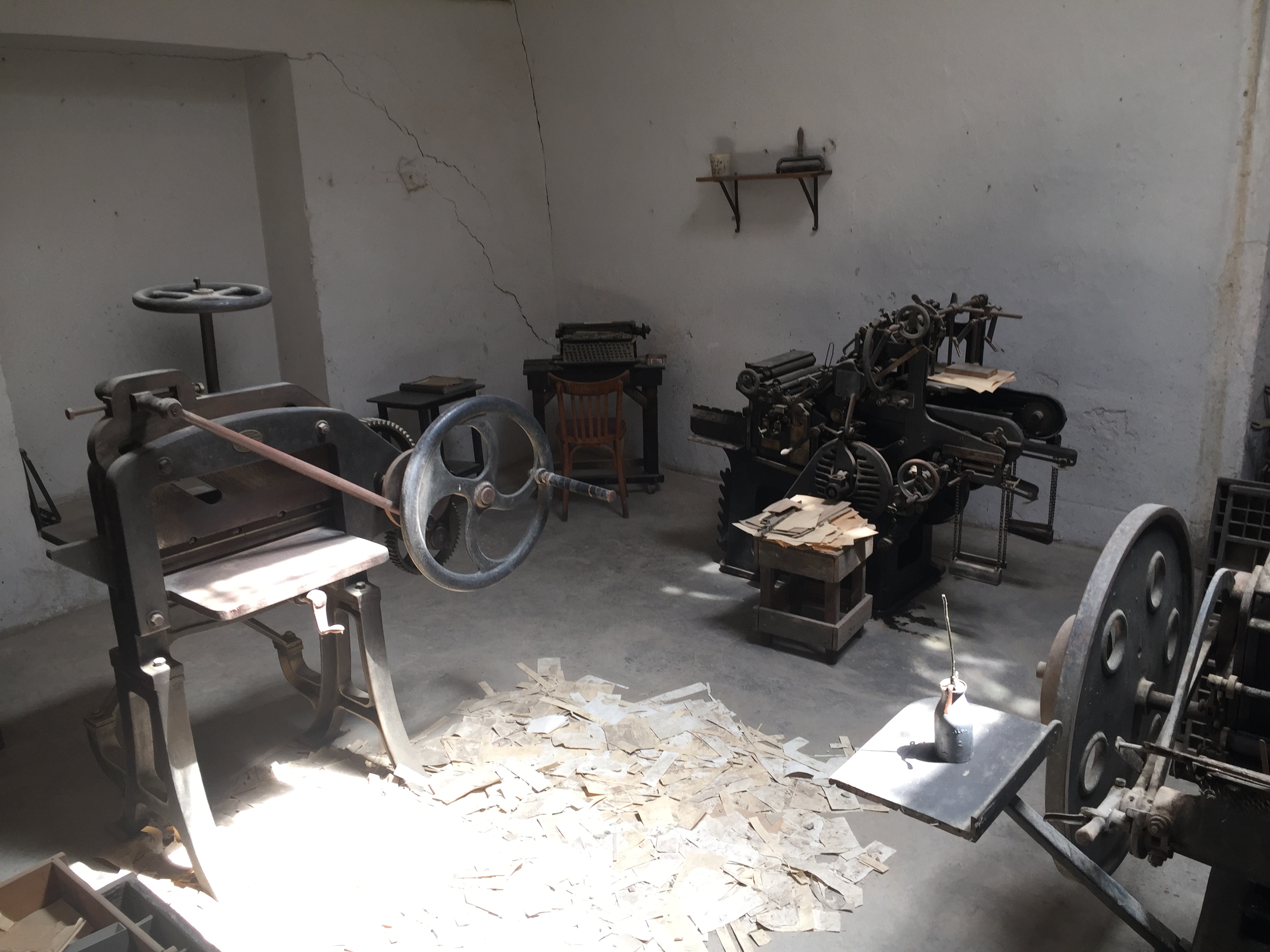The photograph captures an indoor scene of an old, possibly manually operated workshop, featuring a variety of intricate machinery. The left side of the image showcases a machine with two prominent wheels and a long metal bar, raised on metallic legs. Below this apparatus lies a scattered pile of shredded paper, partially illuminated by sunlight. A small, simple desk, complete with a typewriter and a diminutive wooden chair, occupies the corner of the room. There is also a coffee table with a book atop it and a shelf mounted on the white, cracked wall. The backdrop reveals an aged printing press, compact enough to fit inside a truck, characterized by numerous gears and pulleys. The machinery throughout the room hints at a bygone era of manual operation, further emphasizing the workshop’s nostalgic charm.